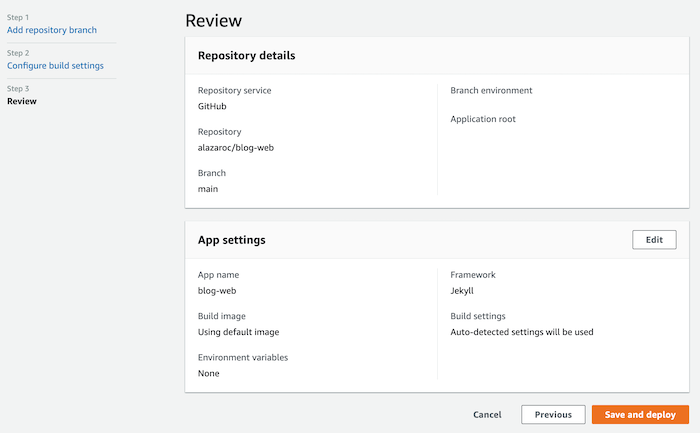Detailed Caption:  
The screenshot displays a GitHub repository page showcasing the configuration and review process for deploying an application. The page is divided into three primary steps, mentioned at the top of the page:

1. **Add Repository Branch**: Highlighted in blue, located on the upper left-hand side.
2. **Configure Build Settings**: Presented in gray, followed by blue text.
3. **Review**: Indicated in black, marking the current step.

Below these steps, the page details the repository settings under the heading "Review Repository Details" in bold black text. The comprehensive details are as follows:

- **Repository Service**: GitHub
- **Branch**: Main
- **Environment**: Application root
- **Repository**: azalarkblog.web
- **App Settings**: Editable via a button on the far right
  - **App Name**: Blog web
  - **Framework**: Jekyll
  - **Build Image**: Default image
  - **Build Settings**: Auto-detect settings will be used
  - **Environment Variables**: None specified

At the bottom of the page, there are three actionable buttons: 
- **Cancel**: Standard button.
- **Previous**: Displayed in a white box with black text.
- **Save and Deploy**: Highlighted in an orange box with white text, indicating the action to finalize and deploy the configurations.

This GitHub repository page is designed for users to manage and deploy their open-source applications, demonstrating the configuration specifics for the "azalarkblog.web" application using Jekyll as the framework.